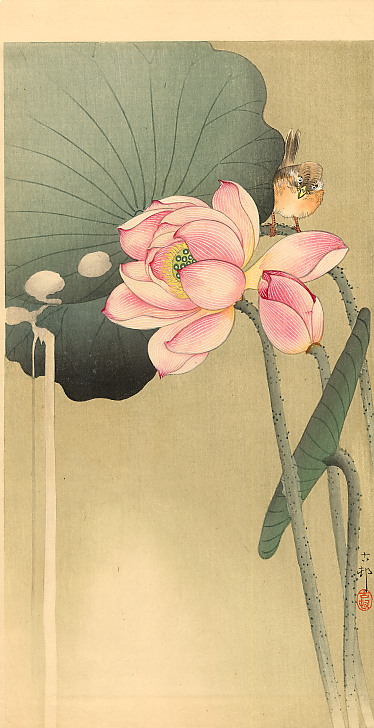This artwork, possibly a Japanese painting, vividly illustrates a serene natural scene. At the center, a pink lotus blossom with green circles and a yellow center unfurls its delicate petals. The flower, set against a backdrop of large green leaves, displays intricate details including darker green dots that texture its light green stem. Atop the tall, knobbly stem, a small bird perches gracefully. The bird, resembling a finch or songbird, boasts a peachy-pink chest, a tan head, and a brown back and tail, with white markings around its eyes and a yellow bill. The scene is completed with dewdrops or a creamy substance dripping from the leaf, adding a sense of freshness. The background is a light cream color, aged to a yellowish hue. In the bottom right corner, a red and black symbol, possibly Japanese writing, stands out, enhancing the painting's authenticity and suggesting its Asian origin.